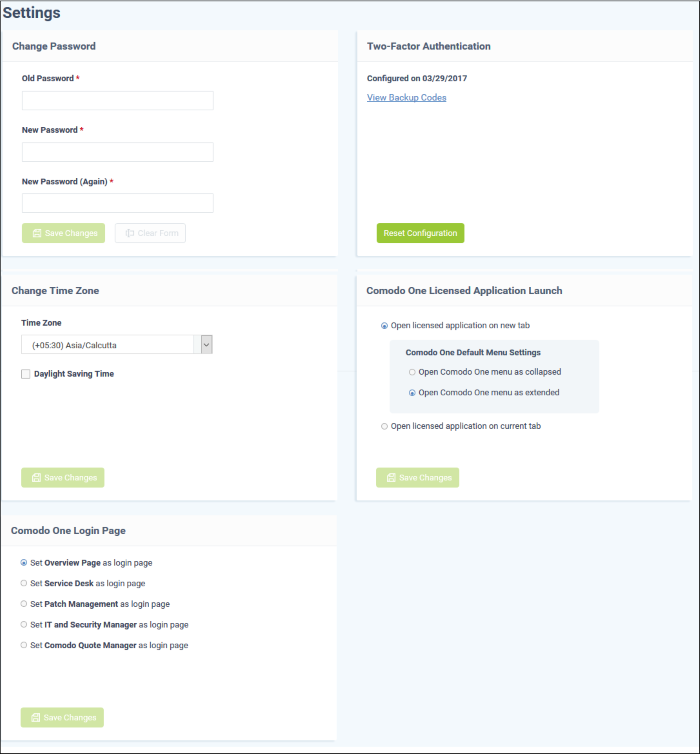Detailed Caption:

The image showcases a comprehensive settings page for a web service or application, primarily focused on user account management. The page is systematically divided into five main sections:

1. **Change Password**: This section includes fields for entering the old password, the new password, and a confirmation field likely for re-entering the new password. At the bottom of the section, there are "Save" and "Clear" buttons for applying or discarding the changes.

2. **Two-Factor Authentication**: This area displays the configuration date for the two-factor authentication setup and offers backup codes to reset the configuration if needed.

3. **Change Time Zone**: Featuring a dropdown menu for users to select their preferred time zone, this section also includes an option to enable or disable daylight savings time. A "Save" button is provided to save any changes made.

4. **Komodo One Licensed Application Launch**: This section allows users to modify how the Komodo One application launches. Options may include settings for whether the interface starts in a collapsed or extended state, among other customizable settings.

5. **Komodo One Login Page**: This area is likely focused on settings related to the login interface of the Komodo One application.

The settings page is designed with a user-friendly layout, ensuring all crucial account management functions are easily accessible and configurable.